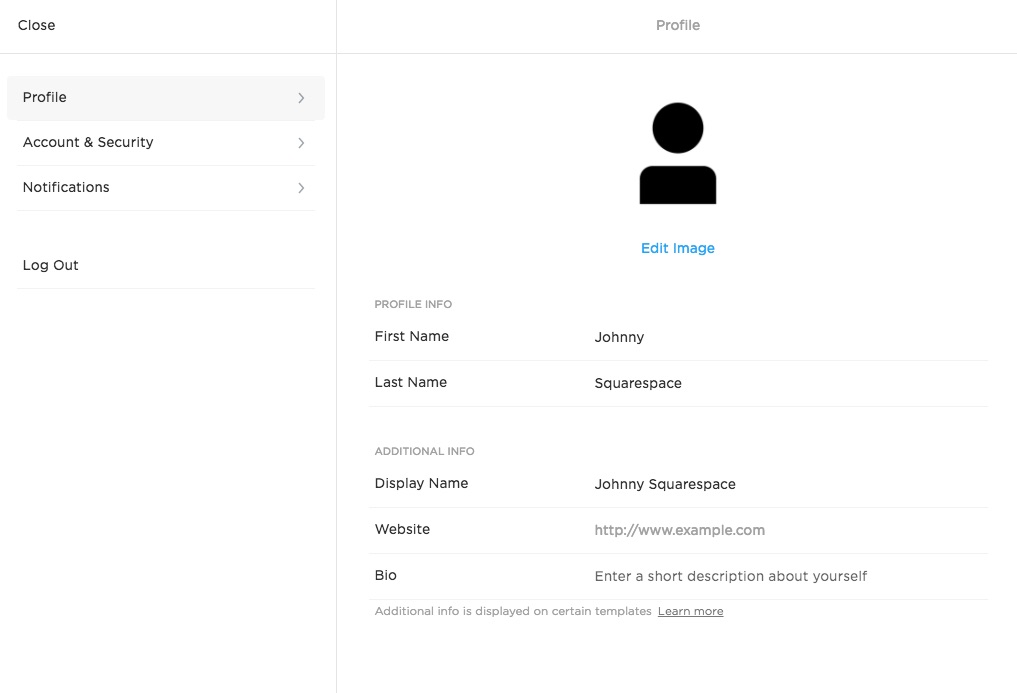This image depicts a profile page on a website with a minimalist design and a monochromatic color scheme, featuring gray and black text on a white background. At the top of the page, the word "Profile" is prominently displayed. Below the title is a gray navigation bar.

On the left-hand side of the page, there is a sidebar with several options: "Close" at the top, followed by "Profile," which is highlighted in gray, "Account and Security," "Notifications," and "Log Out."

The main body of the page includes a profile section. At the top of this section is an image placeholder for a person's profile picture, showing both the head and upper body. Beneath this image is a blue link labeled "Edit Image."

The profile information is listed in a form-like manner:
- First Name: Johnny
- Last Name: Squarespace
- Display Name: Johnny Squarespace
- Website: www.example.com

Following the website field is a "Bio" section, prompting the user to "Enter a short description about yourself." Below this bio field is a note stating, "Additional info is displayed on certain templates," with a "Learn More" link that is underlined and highlighted in gray.

The overall design of the website is very clean and simple, with no distracting colors or flashy visuals, focusing purely on text and basic navigation elements.